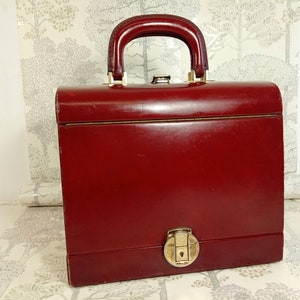The image depicts a square-shaped, red leather bag with two handles, designed in the style of a briefcase. The leather has a low luster, indicating it is not new but still in good condition. The bag features gold or brass fittings, including a circular latch at the front and another small latch under the handle, which appear slightly eroded or rusted with time. Accentuated with pink or gold highlights, the bag exudes an expensive and vintage aura. The backdrop showcases a delicate, flowery white wallpaper patterned with light gray trees and leaves, resembling Japanese line art on an egg-colored background. The detailed and slightly worn aesthetic of both the bag and the background suggests the photo might be intended for an online marketplace, like eBay.